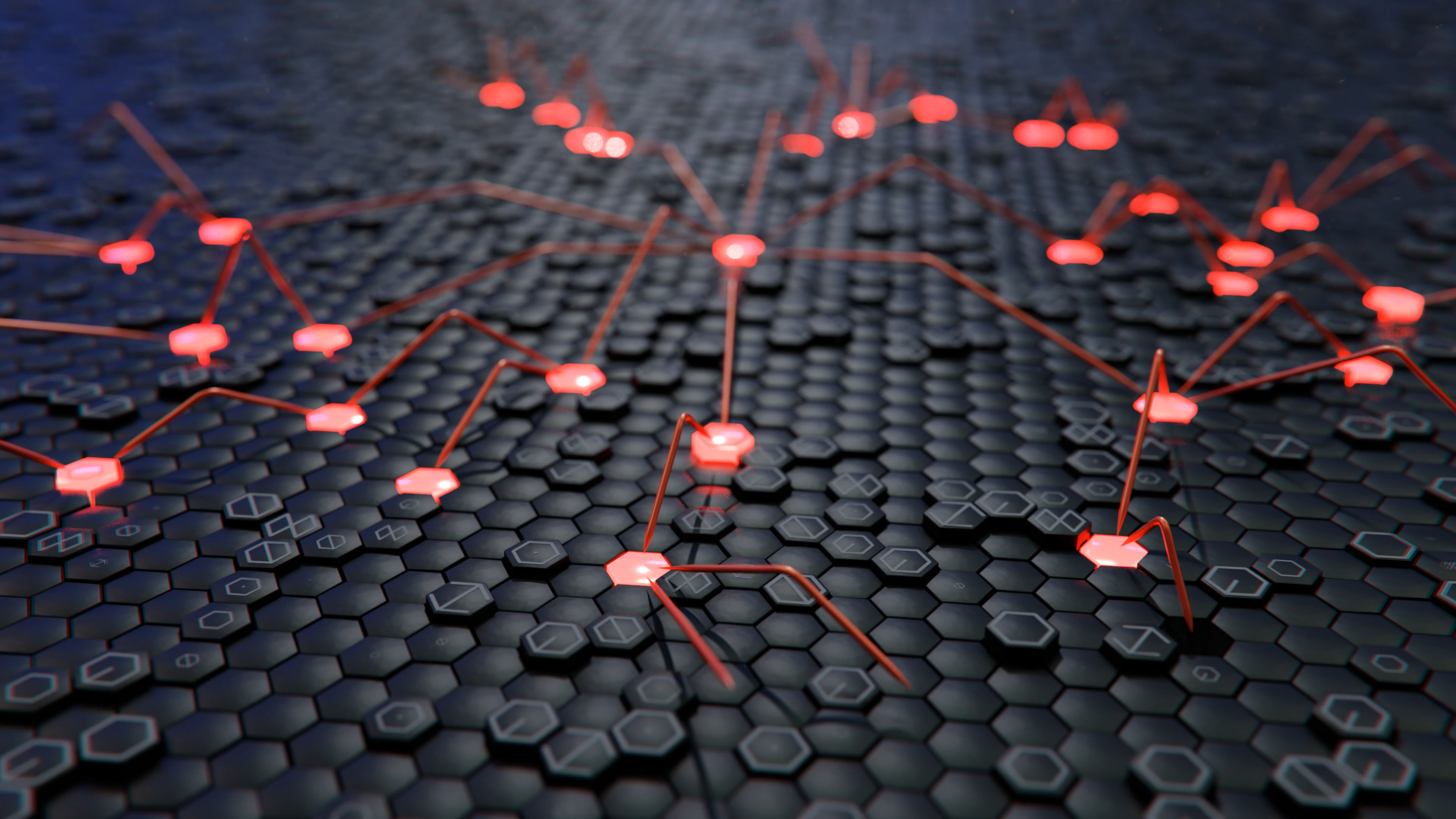The image is a detailed, wide horizontal digital depiction resembling a densely packed circuit board with a vast honeycomb pattern. Each cell within the pattern is octagonal, resembling tiny stop signs, and they are arranged in very tight horizontal rows. The surface is visually textured, as some of the octagons are smooth while others are raised, creating an undulating effect. Throughout the image, a few of these octagonal cells are illuminated with a fluorescent red glow, giving them a striking contrast against the black background. These glowing cells have thin, spindly red wires extending from their edges, mimicking the appearance of electric spiders with legs that arch out and then slant back down towards the surface, forming a web-like network. Additionally, some of the non-glowing cells are intricately detailed with fine gray lines that outline their shapes or dissect them, enhancing their structural appearance. As the view progresses towards the top, the image blurs slightly, giving a sense of depth and distance, but the consistent honeycomb pattern persists throughout.